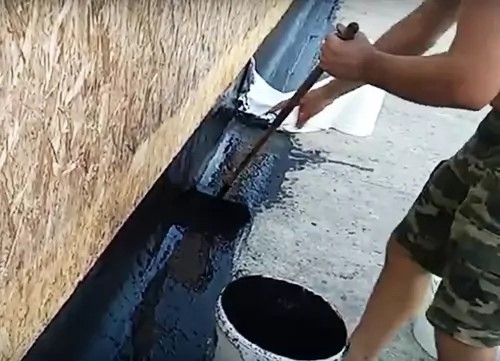In the image, a Caucasian individual is wearing green and light-green khaki shorts, standing on a grey concrete floor. They are next to a plywood wall with varying shades of light and dark brown. By their foot, there is a white bucket containing a black substance, likely tar. The person is holding a broom and is in the process of spreading the black tar on the base where the foundation meets the concrete floor. Behind them, between their legs, is another white bucket. To the right, a white sheet of paper is positioned, possibly as a guide indicating where the tar needs to be applied. The black tar has already been spread along the base, as evidenced by the visible marks on the wall and floor.